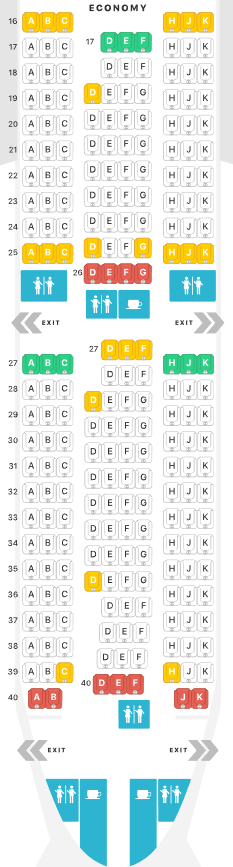The image is a detailed seating chart of an airplane, characterized by sections of organized seating arrangements and a variety of symbols.

Starting from the left side of the chart, there is a gray line marking seats numbered 15 to 21. Adjacent to this, a white line features seats numbered 22 to 40. This line is predominantly labeled "Economy."

The seating arrangement includes two rows on one side, colored in yellow with seats labeled ABC ABC. The remaining seats along this section are predominantly white and black, interspersed with blue and white icons representing people. Additionally, there is a coffee cup icon in blue and white.

To the right, a row of seats features three green seats, three gold seats, and four red seats, followed by more blue and white icons representing people, and another coffee cup icon. Further along, six gold seats continue the pattern before transitioning to more white and black seats.

Notable symbols such as blue and white icons representing people and gray arrows indicating exits appear on both sides of these seat rows. Continuing down, there are six green seats, approximately seven gold seats, and around seven red seats interspersed with a greater number of white and black seats.

Towards the bottom, blue and white icons representing people appear again on either side, along with two more coffee cup icons. Lastly, the chart features additional gray arrows marking exits.

Overall, the chart is a comprehensive and visually diverse representation of airplane seating, highlighting various seat sections and important icons for passengers.